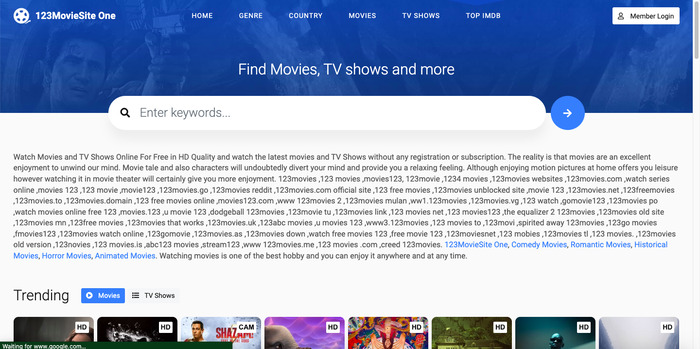This horizontal screenshot captures part of a movie website interface, specifically "123 Movie Site 1," prominently positioned at the top left in neat, bold letters. Adjacent to the site's name is a white circular icon resembling a film reel, adding a classic cinematic touch. The navigation bar just below features six drop-down menus labeled Home, Genre, Country, Movies, TV Shows, and Top IMDB, offering users a seamless browsing experience. 

In the upper right corner, a white Member Login button stands out against the site’s blue, translucent banner. The banner itself subtly displays the image of a man on the left, adding depth and visual interest. Beneath this banner, a long white search box invites users to "Enter Keywords," accompanied by a blue arrow icon suggesting ease of access for search functionality.

Following the search box, an extensive textual section emphasizes the site’s branding with frequent mentions of "123." This text likely hints at possible search terms and themes for user convenience. Embedded within this text are highlighted blue links, directing users to specific categories such as Comedy Movies, Romantic Movies, Historical Movies, Horror Movies, and Animated Movies, with a repeated emphasis on "123 Movie Site 1."

At the bottom, although partly clipped off, lies the Trending section. This includes a blue-highlighted button labeled Movies, flanked by another button labeled TV Shows. The Movies button is activated, showcasing eight cropped movie thumbnails marked either HD or CAM, indicating the quality and type of the available streams.